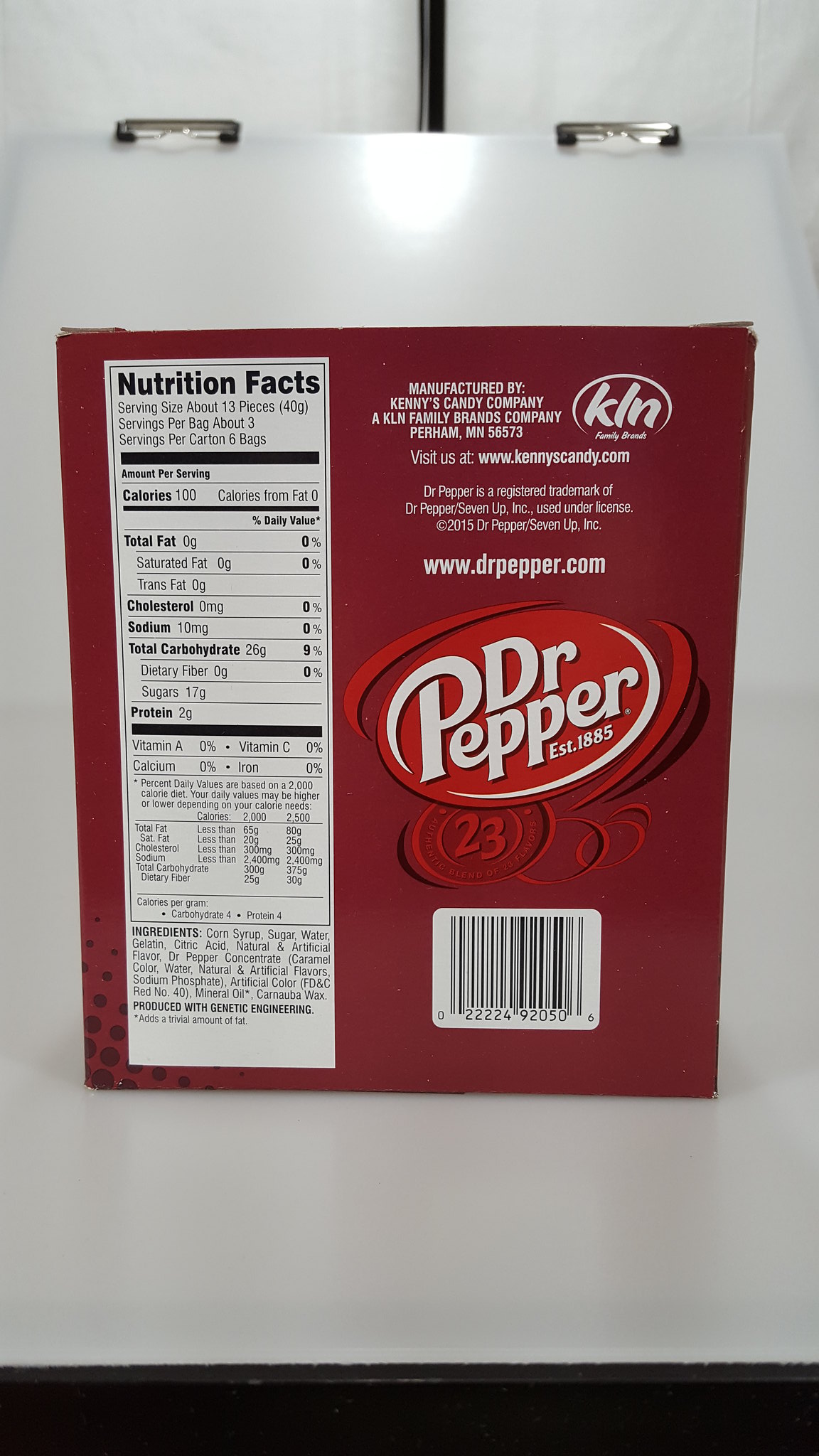The image shows the back of a burgundy-colored Dr. Pepper themed box, possibly a cardboard case or a 12-pack, prominently displaying the Dr. Pepper logo in bright red. The box is situated on a white table, which makes it stand out clearly. Along the left side, there's a long, unreadable nutrition facts label. The packaging indicates it's a snack or candy item, perhaps gummy snacks, as the nutrition facts mention a serving size of 13 pieces, around 3 servings per bag, and 6 bags per carton. Ingredients listed include corn syrup, sugar, water, gelatin, and natural and artificial flavors. Also visible is a logo mentioning "KLN" and an estimated establishment year of 1885.